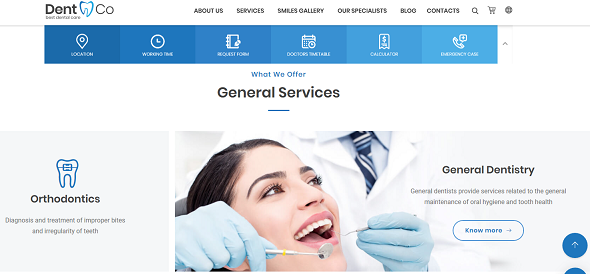In the image, the header displays the name "Dent Co" at the top left, accompanied by a blue tooth icon next to the text "Dent Co" written in black. The header also contains navigation tabs in black against a white background, which include: About Us, Services, Smiles Gallery, Our Back List, Our Special List, Blog, Contact, and a Search icon.

Below the main menu, there is a secondary menu comprising blue tabs with white text. The tabs are labeled: Location, Working Time, Request Form, Donors, Timetable, Calculator, and The Call.

Underneath these menus, the heading "What We Offer" is prominently displayed in blue text. Following this, a subheading "General Services" is written in black.

In the lower left corner of the image, there is a small grey section featuring a blue tooth icon and text describing "Autodontics," which refers to the diagnosis and treatment of improper bites and teeth irregularities.

On the right side of the image, there is a section showing a doctor in a white coat and blue gloves treating a patient's teeth, accompanied by the title "General Dentistry." This section explains that general dentists provide services related to the overall maintenance of oral hygiene and dental health. At the bottom, there is a blue button labeled "Know More."